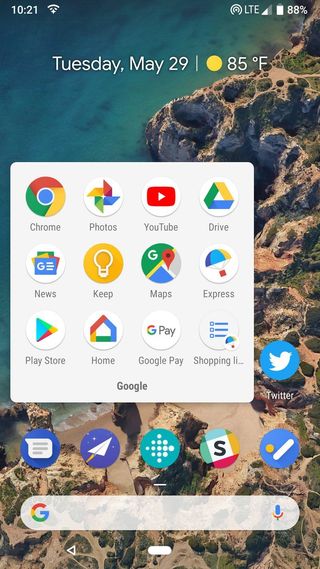The image depicts a mobile phone screen with a serene underwater coral reef screensaver. The screensaver showcases a variety of dead coral formations, with the water surrounding them displaying a vibrant mix of blue and green hues. In the center of the screen, there is a white square containing several application icons arranged in a grid. These icons include recognizable Google services such as Chrome, Photos, YouTube, Drive, Express, Maps, Keep, News, Play Store, Home, and Google Shopping Lists. To the right of this grid, the distinctive blue Twitter icon is prominently displayed over the screensaver. Scattered around the screen are additional app icons, some of which are unidentifiable, except for one featuring a pencil and a yellow dot, indicative of a note-taking application. The search bar at the bottom of the screen remains empty, suggesting no active queries or selections.